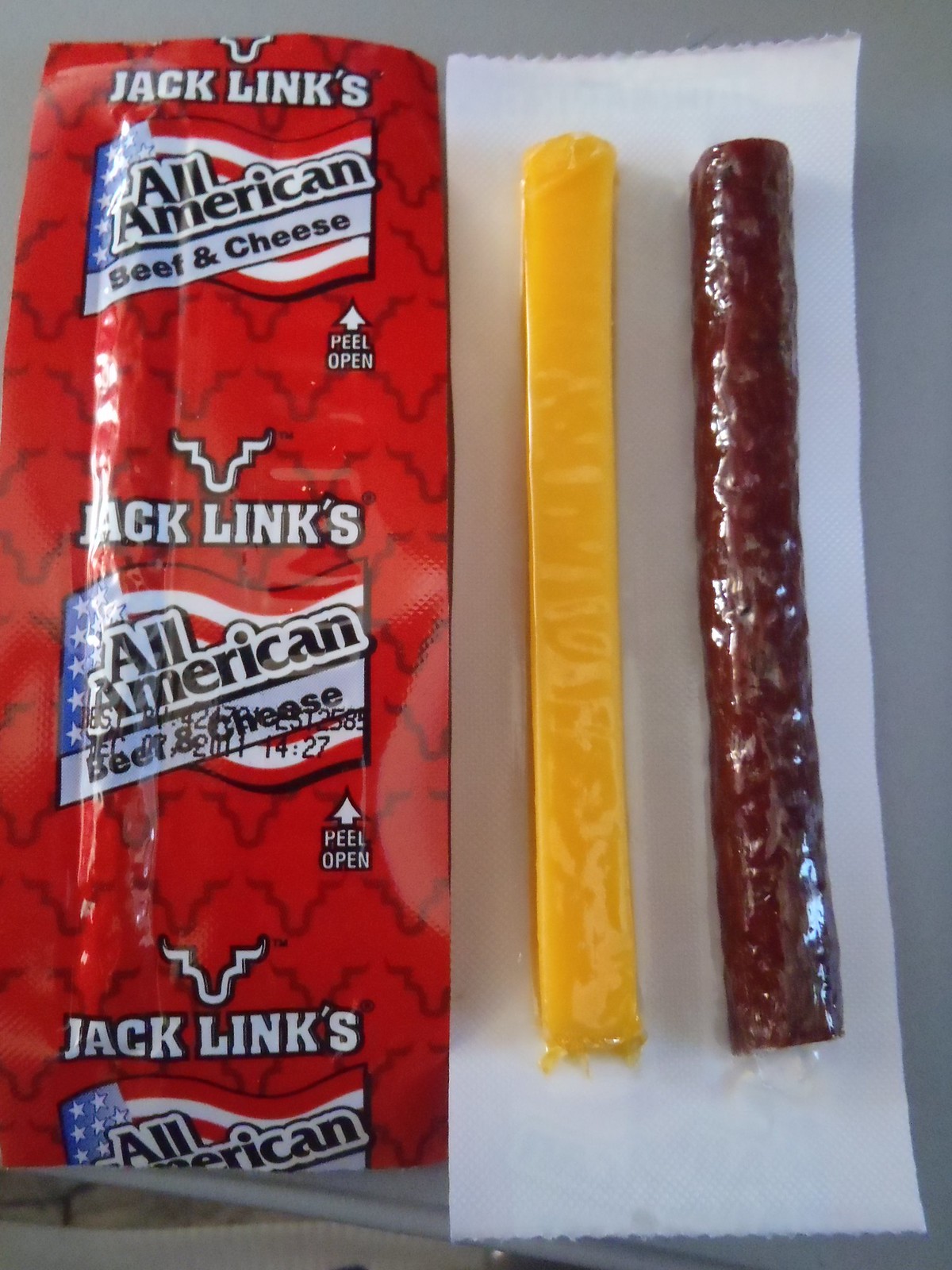The image showcases a package of Jack Link's beef and cheese snacks displayed on a gray countertop. On the left side of the image sits the red-colored wrapper featuring the "Jack Link's" brand name in white text repeatedly, and prominently displaying a logo resembling an outline of a cow's head minus the top portion. The wrapper also highlights the product as "All American Beef and Cheese" in black text on a white background set against an American flag motif. On the right side, removed from the wrapper, lies the actual product: a thin, yellowish-orange stick of cheddar cheese encased in clear plastic alongside a reddish-brown cylindrical beef stick, also encased in clear plastic. Both items together represent the quintessential beef and cheese snack combo.